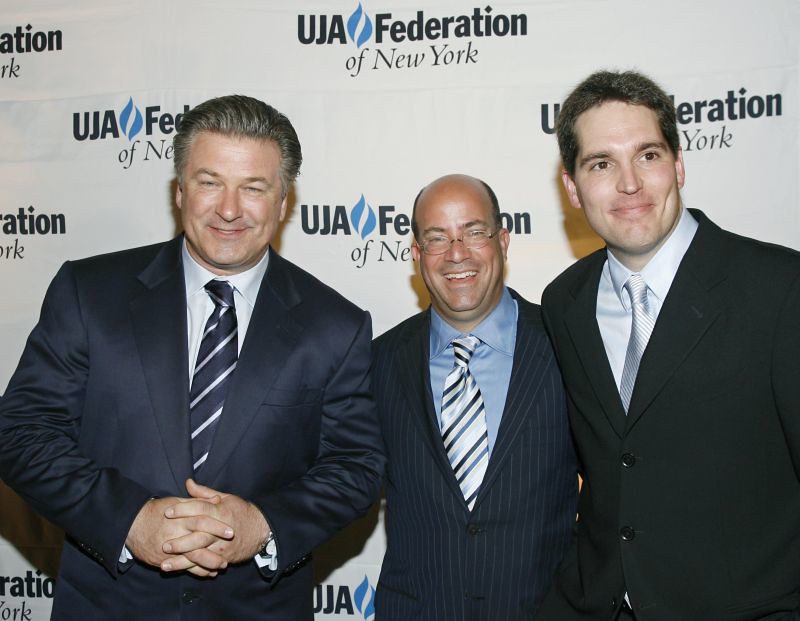This photograph captures three men in formal attire at a fundraising event, set against a press wall adorned with the "UJA Federation of New York" logo on a white backdrop. On the left stands Alec Baldwin, the renowned actor, smartly dressed in a dark blue suit, a white shirt, and a blue, white, and gray striped tie. He has salt-and-pepper hair neatly combed back and is smiling with his hands clasped in front of his stomach. The middle figure is a shorter, balding man with a pronounced tan, sporting glasses, a dark blue pinstriped suit, a blue button-down shirt, and a blue, dark blue, and white tie, suggesting he might be an executive. On the right, a younger man with short brown hair and brown eyes appears, wearing a black blazer, a white shirt, and a light-colored tie. All three men, who are smiling, seem pleased to be at the event, their dark-colored suits contributing to the formal atmosphere.